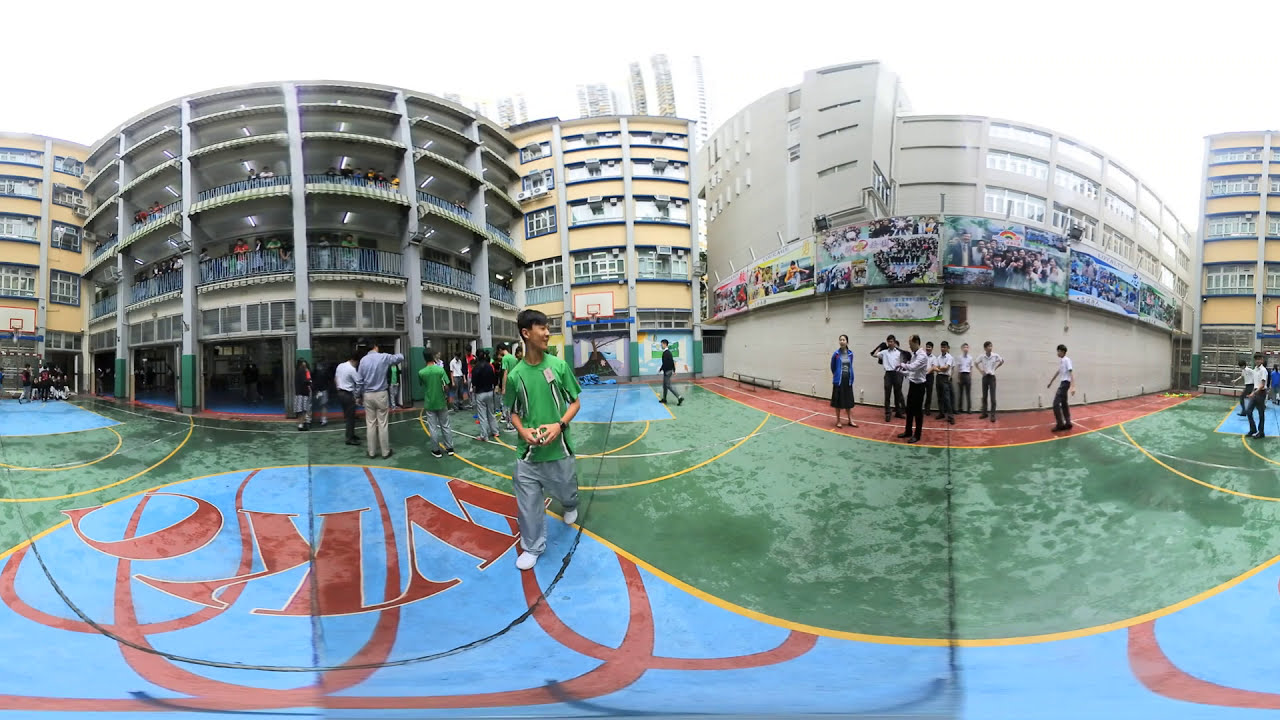This is a highly detailed, 360-degree panoramic image of a bustling school courtyard featuring a full basketball court adorned with vibrant colors. The court itself is primarily blue with yellow markings for the top of the key and the three-point line, and a distinctive "WKC" logo in red sits at center court amidst several red lines. Positioned centrally within the image is a young boy wearing gray pants and a green shirt, looking to his left while holding an unidentified object. Surrounding him, numerous school children in matching black pants and white shirts, likely school uniforms, are engaged in various activities. The scene is framed by multi-story buildings with balconies, suggesting a school complex with attached residential units or perhaps teacher accommodations. The buildings feature numerous window air conditioners and a prominent mural on one side. The courtyard appears wet, indicating recent rain or ongoing cleaning, and another basketball hoop is visible above the boy's head, implying multiple courts in the vicinity. The atmosphere is lively with both students and teachers interacting, and it seems like a vibrant moment captured during a school event or break time.